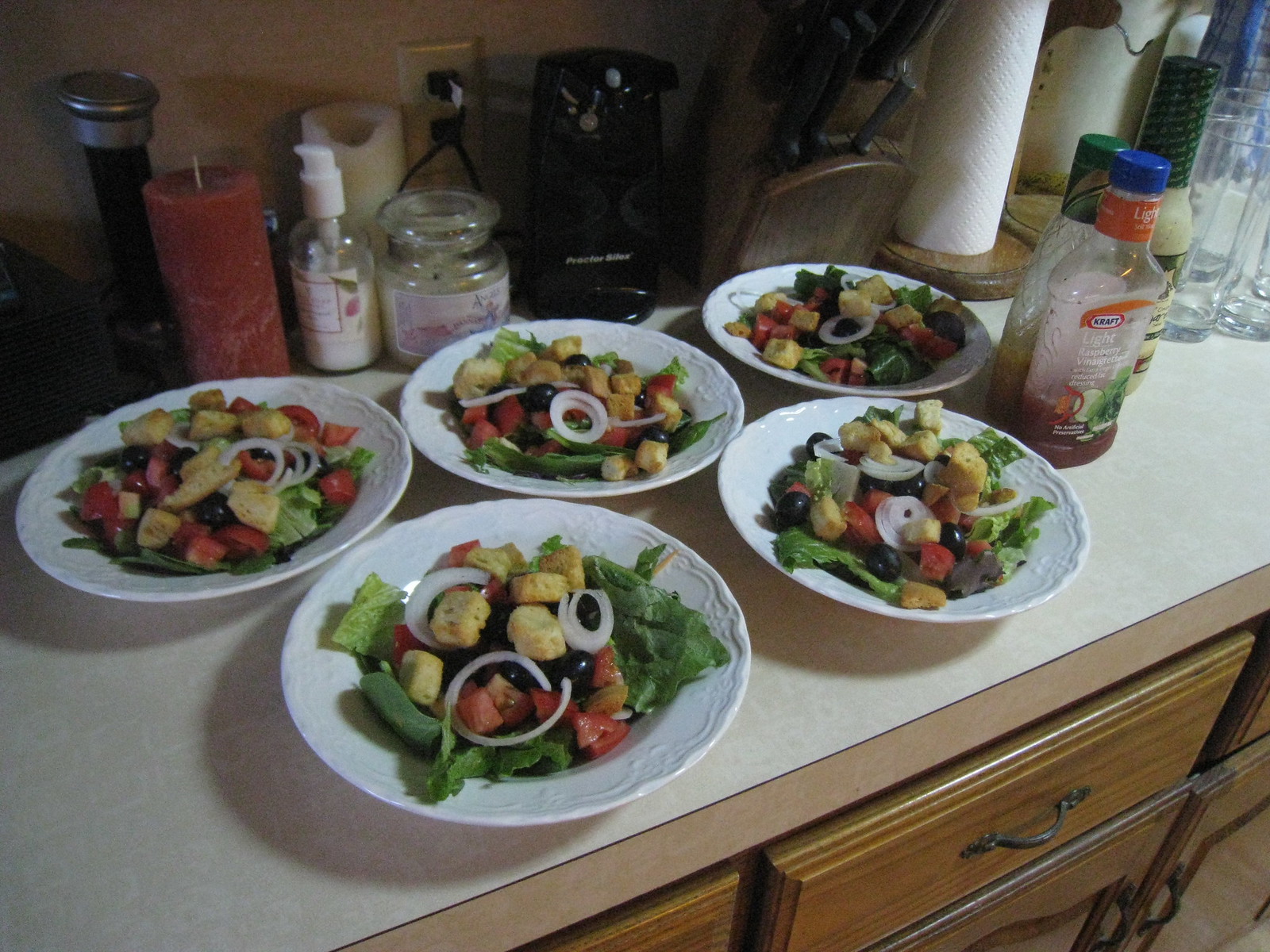The image depicts a kitchen countertop laden with five meticulously prepared salads, each on a pristine white plate. The salads, arranged in a staggered, pyramid-like formation with three plates at the back and two at the front, comprise fresh green lettuce, sliced onions, vibrant tomatoes, savory black olives, and crunchy croutons. A collection of salad dressings, including one from Kraft, is positioned to the right, offering a variety of choices for the upcoming meal. The white countertop is speckled with several other items: a roll of paper towels on a wooden holder, a black electric can opener, a knife block, a pepper mill, and an array of candles—one tall and red, another tall and white, and a shorter one—adding a touch of ambiance. Wood drawers with small pull handles are visible beneath the counter, and a few glass cups are also situated towards the right side, completing the tableau of a well-prepared kitchen scene.